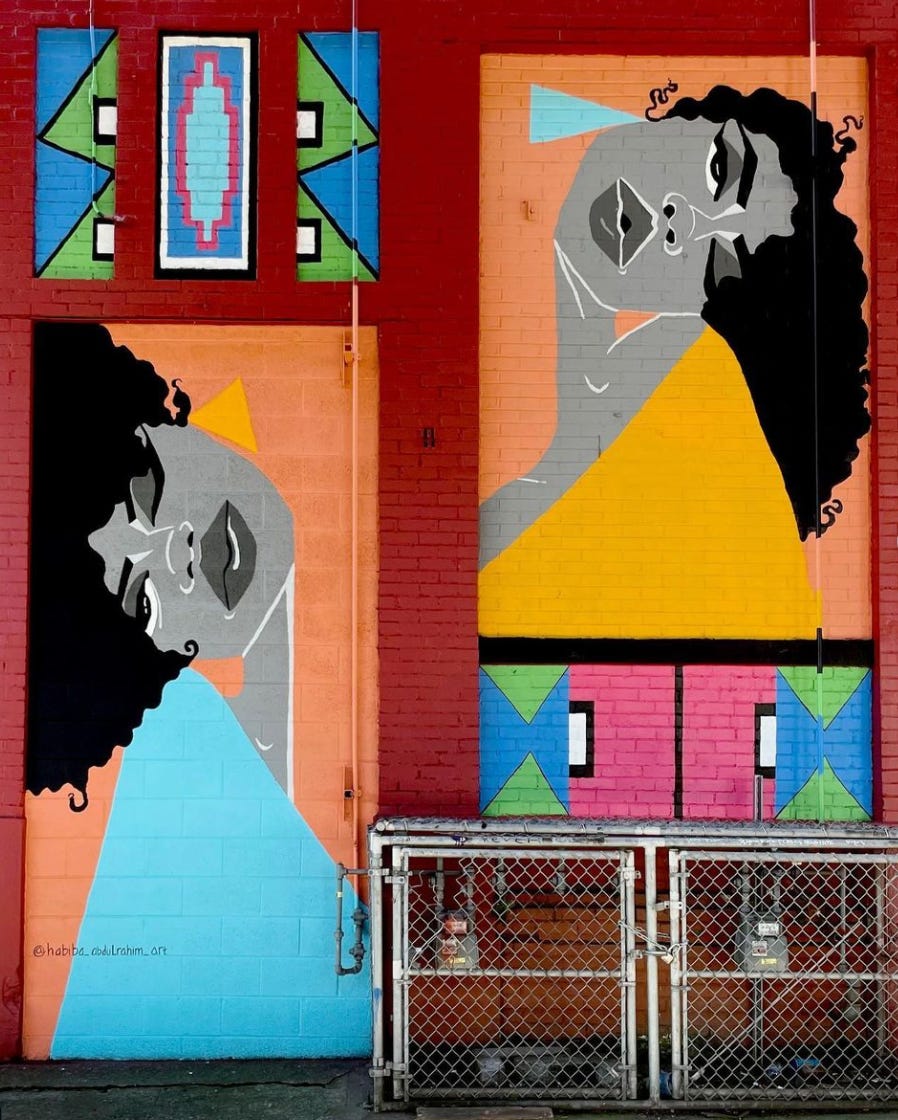The intricate mural on the brick wall features two prominent grayscale portraits of women, each uniquely positioned and stylistically distinct. The first portrait, located in the upper right corner, showcases a woman's face turned sideways to the right. This woman has gray skin with darker gray lips; her expressive eyes feature one that is open and one that is almost closed, barely revealing the top line of her pupil. Her curly hair flows elegantly from the top side, cascading nearly halfway down the wall. 

Directly beneath in the bottom left corner, the second portrait depicts another woman, her face turned sideways to the left. Like the first, she has gray skin and darker gray lips, with one eye partially open. However, her hair contrasts sharply as it is styled upwards in a voluminous ball. 

Between these two portraits on the upper left section of the wall are Native American-inspired graphics. One graphic includes a teal-colored center with expanding straight edges. Overlaid across this mural is an array of geometric shapes and vibrant colors, including a blue triangle pointing towards the lower portrait and a green tree-like pattern in the upper left corner.

Dominating the bottom right, two dirty silver chain-link gates form an enclosure, bound by a silver chain and lock, possibly guarding an entranceway into a building. Amidst these gates, additional graphics appear—each with rectangles containing converging triangles and vivid colors—that complement the overall graffiti-esque yet meticulously designed aesthetic of the mural. Lastly, in the very bottom right corner, there's some text likely displaying a social media link for the artist, surrounded by a circular "C" symbol and letters, "H-A-B-T-B-A dot C-D-U-A-R-A-H-M underscore O-R-T."

The mural, richly detailed and visually compelling, transforms the dark red brick wall into a vibrant canvas, seamlessly blending artistic expression with urban elements.